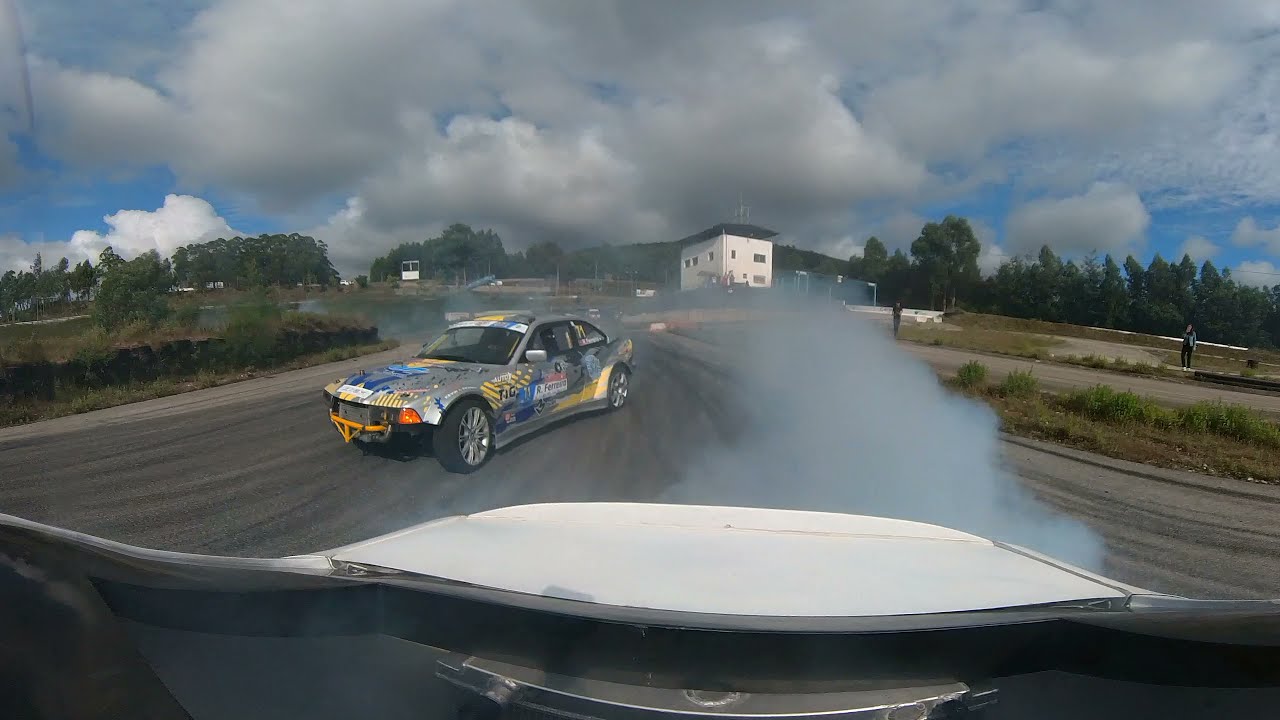Captured from within a white rally car during a high-speed race, this dynamic image uses a fisheye lens to enhance the scene's intensity and distortion. The perspective is through the back window, highlighting a following gray rally car adorned with blue and yellow decals and missing its front bumper. Thick smoke, possibly from the tires or exhaust, billows from the trailing car, adding to the sense of speed and power. The race is set on a blacktop track lined with greenery and scattered spectators, including a woman in a jean jacket and black pants. In the background, a prominent white building with several windows stands out against a vivid blue sky filled with large, fluffy clouds. Trees and other foliage frame the horizon, emphasizing the outdoor setting and creating a picturesque backdrop for the thrilling race.